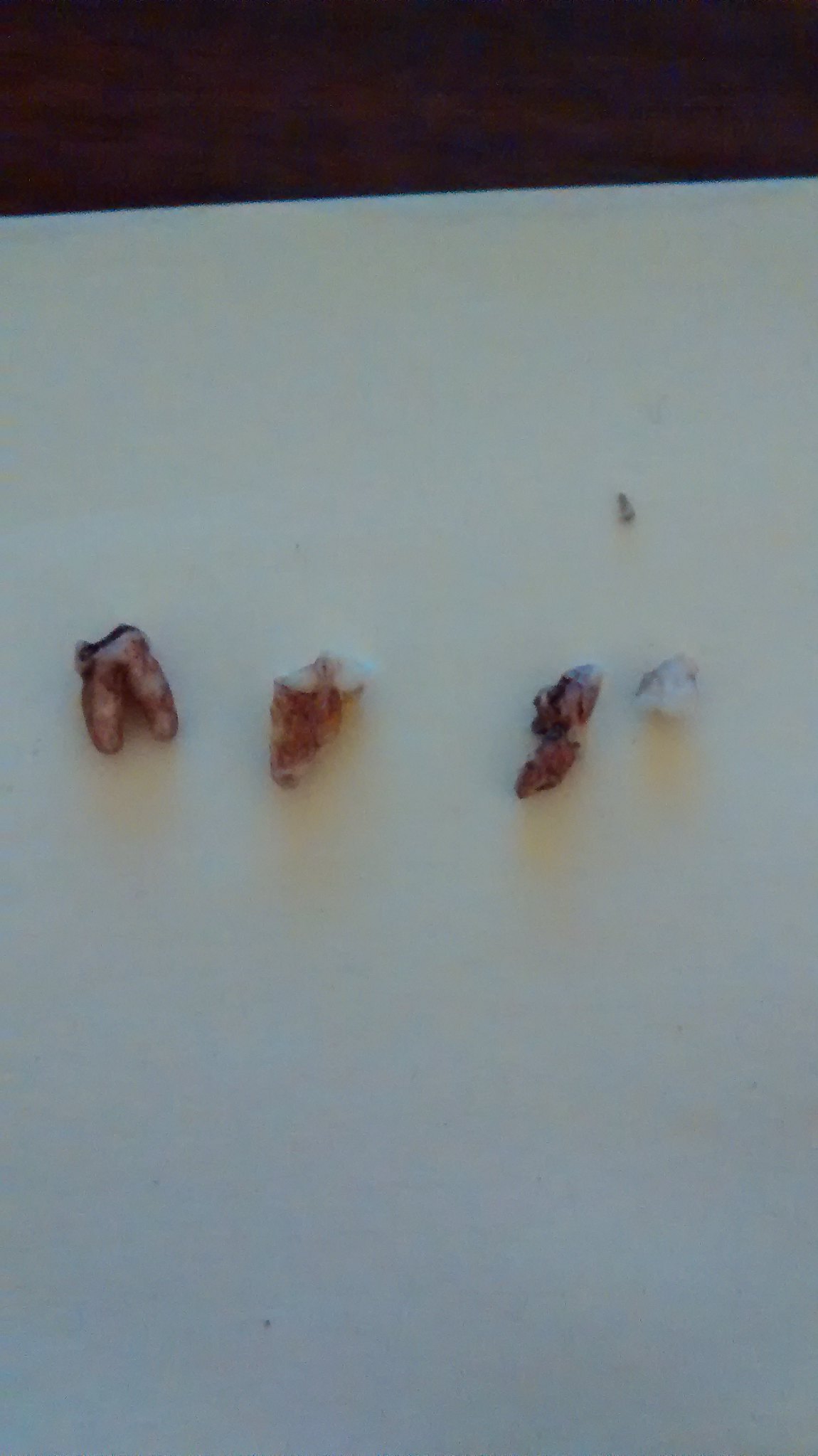The photograph depicts a white plate lying on a white surface, showcasing a stark contrast against a black background at the top. Four objects resembling rotten teeth and teeth fragments are meticulously arranged horizontally across the middle of the plate. The leftmost object appears to be a tooth with two prongs, characterized by a pale white color marred with brown stains and a black, decayed crown. Adjacent to it is a fragment with a jagged top, featuring a black and white hue with brown discoloration. The third item in line is another fragment, seemingly broken bones, displaying dark red and black hues with traces of white. The rightmost object is a small, clear and opaque pebble-like piece with white, red, and black cracks. The grotesque display emphasizes the bloody and decayed nature of the teeth fragments, suggesting they are human in origin.